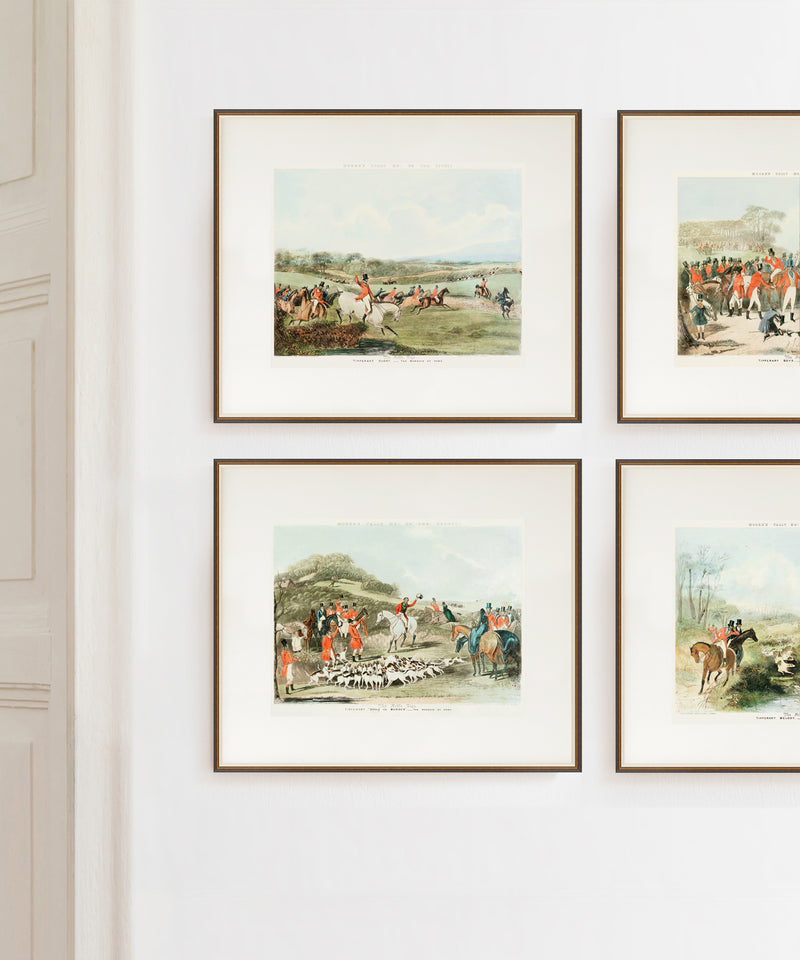The photograph showcases a section of a white wall adorned with four framed prints arranged in a rectangular pattern, equidistantly spaced apart. The prints, bordered by thin black frames and tan-colored mats, depict vintage scenes reminiscent of the 1700s or 1800s. They capture the essence of an old-fashioned fox hunt or hunting expedition, featuring horsemen clad in bright reddish-orange coats and black top hats. 

In the top left print, an action-packed scene unfolds with horsemen gathered, likely preparing for a hunt. Below this, the bottom left print depicts a tranquil hilltop with a flock of sheep, alongside riders and dogs gearing up for the chase. The upper right print, partially visible, continues the hunting theme with detailed figures on horseback. The bottom right print, also partially visible, shows riders by a lakeside, hinting at the continuity of the hunt, with a bird soaring above the brush in the foreground.

To the left of the framed prints, part of a white wooden doorway and some crown molding are visible, adding context to the setting within a home or gallery space. The careful arrangement and historic theme create a cohesive visual narrative of equestrian and hunting traditions.